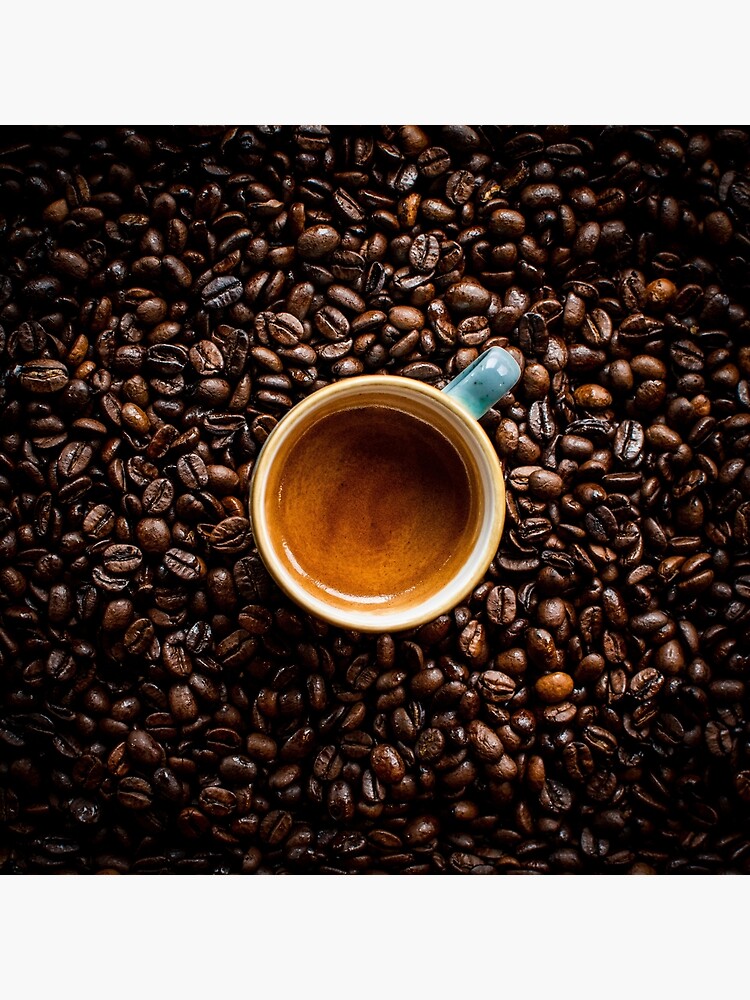This is an aerial, contemporary photograph focused on a coffee mug, ideal for coffee lovers. The entire background is composed of a detailed pile of coffee beans, arranged in such a way that the image forms a perfect square. The brightness of the image transitions from darker on the edges to lighter towards the center, creating a gradient that highlights the rich texture and varied directions of the coffee beans. 

In the very center of this textured backdrop sits a coffee mug, filled with what appears to be espresso. The mug's main body is a creamy yellow color, and its handle transitions from light blue to periwinkle, positioned diagonally from the top left. The coffee inside the mug displays a gradient from dark to light brown, and the interior of the cup appears white against the deep brown of the coffee.

The photograph, taken from above, captures the mug against the coffee beans with precise clarity, showcasing the contrasting shades of brown, light blue, and gold, enhancing the image's artistic and contemporary appeal.